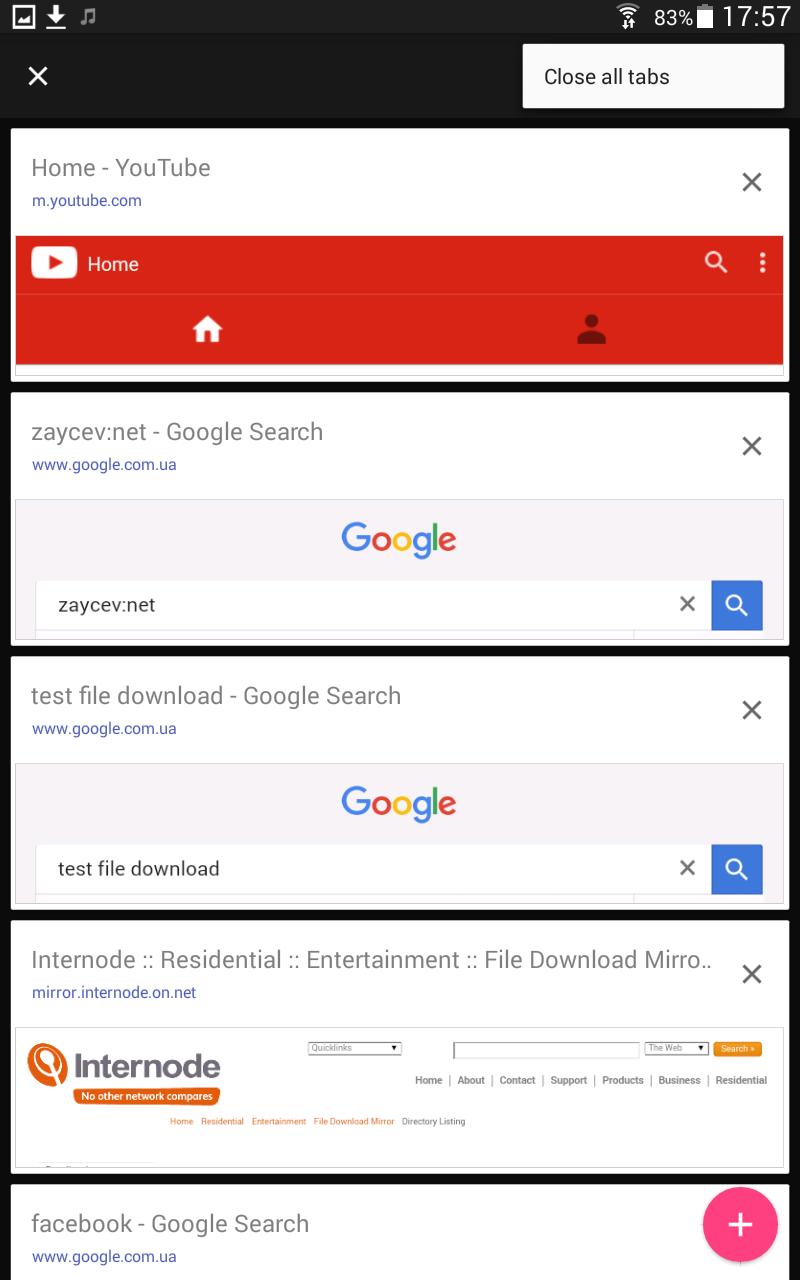This image appears to be of a tablet screen showcasing an array of open tabs and various icons. 

On the left side of the screen, icons for a photo application, download manager, and music player are displayed. On the right side, the status bar indicates that the tablet is connected to Wi-Fi, has 83% of its battery remaining, and the time is 17:57. Below the status bar, on the left, there is an 'X' icon, and on the right, the option to 'Close all tabs' is visible.

The central portion of the screen contains four open tabs represented as horizontal rectangles. The details of each tab are as follows:

1. The top tab is labeled 'Home - YouTube' with the URL 'm.youtube.com'. To the right of this label, an 'X' icon is visible. Below this tab, the YouTube interface reveals a red navigation bar featuring the YouTube logo, a 'Home' button, a profile icon, a search icon, and a vertical three-dot menu icon.

2. The second tab down reads 'zayceb: net - Google Search' with the URL 'google.com.ua'. In the search bar appears 'zayceb: net'. An 'X' icon is located to the right of the search bar, and a blue search button is situated next to it.

3. The third tab reads 'test file down - Google Search' with the URL 'google.com.ua'. The search bar contains 'test file down' with an 'X' icon to its right and a blue search button next to it.

These details collectively paint a comprehensive picture of the contents and layout of the tablet's screen at the moment the image was captured.